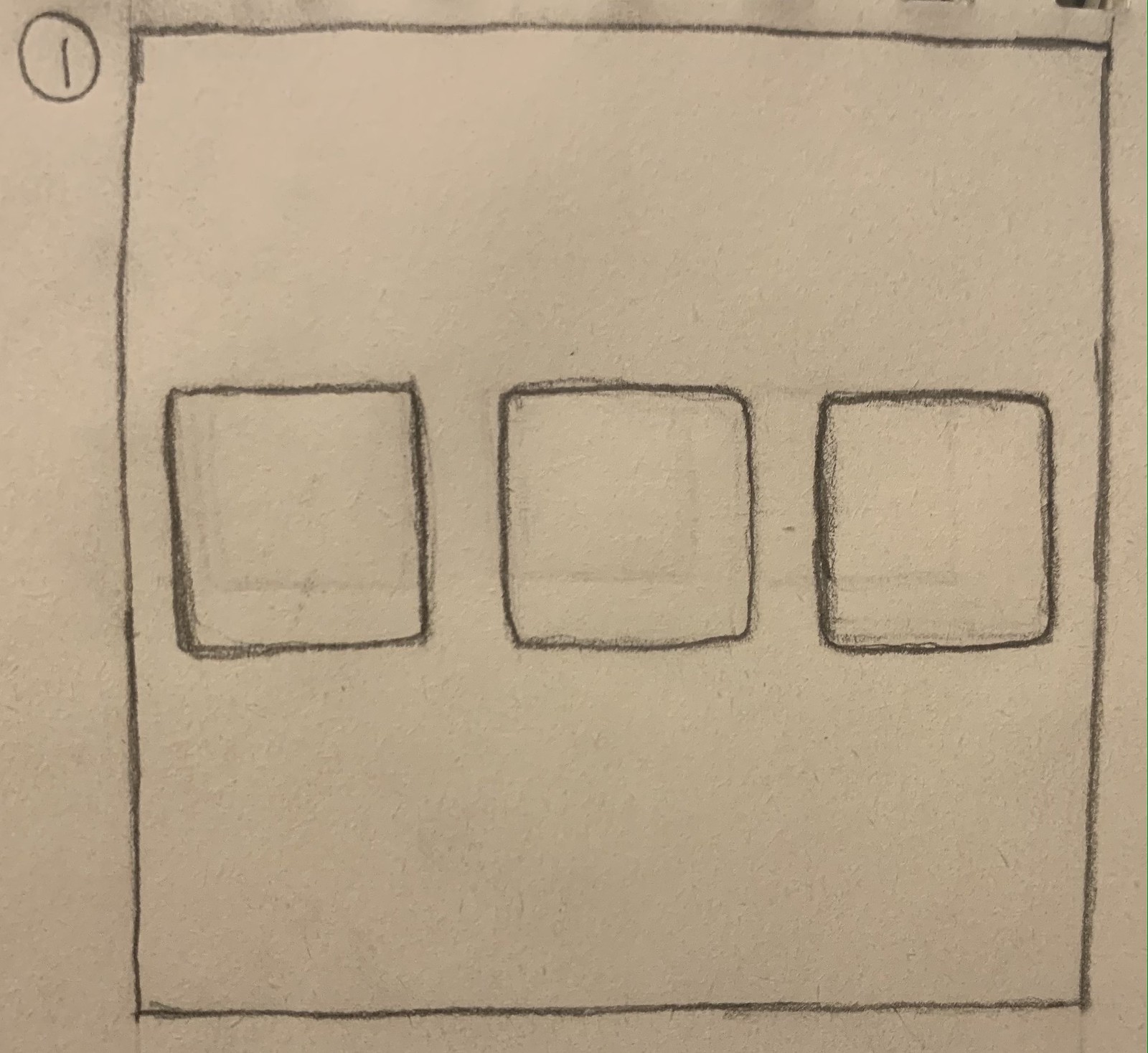The image depicts a simple pencil sketch on a white piece of paper, likely part of a sketch pad. Dominating the drawing is a large two-dimensional square outlined by a single line. Within this square, three smaller squares are arranged horizontally across the center, each featuring light shading along their inner edges. 

In the top left-hand corner of the main square, the numeral "1" is circled. Upon closer inspection, faint hints of other squares and subtle shading can be seen in the background, providing a delicate texture that is easy to overlook. The paper itself has a slightly rough texture, evidenced by small bumps and specks dotting its surface. Additionally, faint gray smudges and a barely noticeable line are present near the top of the page, adding to the sketch's overall simplicity and understated detail.